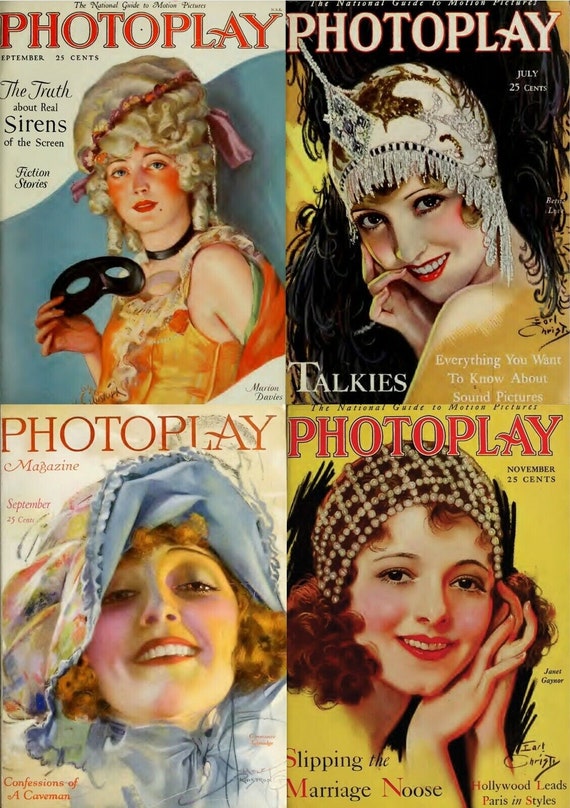This image is a taller-than-wide rectangular composition divided into four sections, each featuring a vintage magazine cover of "Photoplay." Titled "the national guide to motion pictures," each cover, originally priced at 25 cents, showcases a beautifully painted headshot of different women, reflecting an idealized aesthetic with soft features and rosy cheeks. 

At the top left, a woman in a large white wig holds a black masquerade mask, her cheeks heavily rouged and her lips blood-red. She wears a sleeveless dress and stares directly at the viewer, with the magazine cover advertising "the truth about real sirens of the screen."

The top right cover portrays a woman with dark eyes and red lips, smiling with her teeth visible. She wears an ornate, feathery theatre hat, an indicator of the "talkies" era, and the cover teases information about "everything you want to know about sound pictures."

In the bottom left section, another woman, who also smiles toothily, is depicted with short red curly hair and a blue bonnet. Her head is slightly tilted, and she gazes downward towards the viewer, adding a touch of coyness to her expression.

Finally, the bottom right cover shows a woman leaning her hands against her face, smiling gently. She wears an elaborate hat, and an atmosphere of serene elegance radiates from her portrait.

Each cover, marked by the distinct red or white “Photoplay” title, collectively evokes a sense of nostalgic glamour and artistic finesse, characteristic of the early 20th-century cinematic allure.